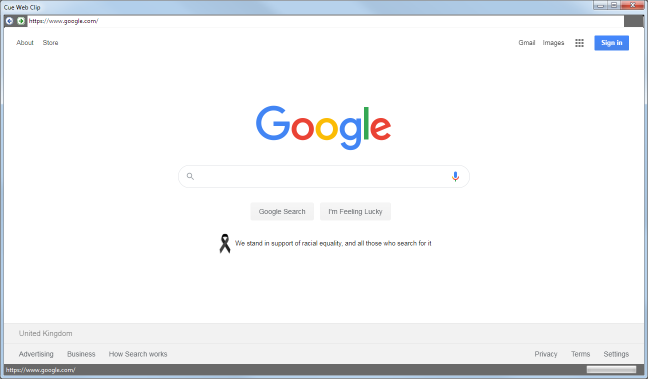The image displays a web browser window with a mix of familiar interface elements and specific details.

At the top left corner of the browser window, there is a blue horizontal band that reads "Queue Web Clip." To the far right of this band, the standard window control buttons are visible: minimize, maximize, and close.

Below the "Queue Web Clip" label, there are navigation buttons; a back button within a blue-outlined white circle featuring a blue left arrow, and a forward button within a green-outlined white circle with a right green arrow. The URL bar shows "https://www.google.com", and underneath it, the text "About Store" is present.

In the center of the page, the Google logo is prominently displayed with its characteristic colors: blue "G," red "O," yellow "O," blue "G," green "L," and red "E." Directly below the logo, there's a search bar containing a magnifying glass icon and a multicolored Google microphone icon for voice search.

Beneath the search bar, there are two buttons: a gray "Google Search" button with dark gray text, and another light gray button with the words "I'm Feeling Lucky" in dark gray text.

At the bottom of this section, a banner reads, "We stand in support of racial equality and all those who search for it."

On the top right of the page, there are links to "Gmail" and "Images." Next to these links, there is a grid icon composed of three squares across by three squares down, forming a larger square. Lastly, there is a blue "Sign in" button indicating the option to log into a Google account.